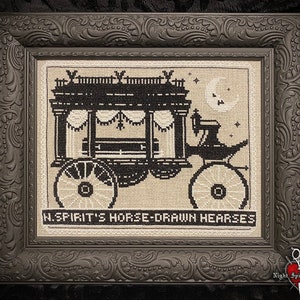This photograph showcases an antique-looking framed print, likely set indoors. The frame, which appears to be crafted from wood or possibly metal, features intricate floral carvings and possibly squirrels, with a flat, dark brown hue. Central to the frame is a brown border enclosing an embroidered print on a light brown or cream-colored fabric. The print itself is black and tan, illustrating a horse-drawn hearse moving towards the right. The hearse, with prominent large wheels, includes elaborate details like windows with white curtains, latticework, and four pillars supporting a roof over a visible coffin. At the driver's section, a sewing machine is depicted. Above this somber scene, a crescent moon and birds (or bats) are present in the top right corner. The bottom of the image features a banner with text in various depictions that reads, "Spirits Horse-Drawn Hearses," with discrepancies in the initials. Additional text, "Z X I G H A," appears in white over a red heart in the bottom right corner. The entire composition exudes an antique, ornate emotion accentuated by the intricate frame and detailed embroidery.